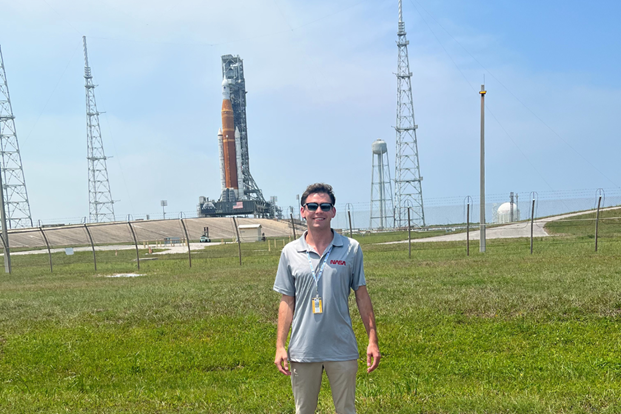The image captures a young white man standing in a green field under a bright blue sky with light, scattered clouds. He is posing for the picture, gazing directly at the camera with sunglasses on his face. He is wearing a gray polo shirt emblazoned with "NASA," a lanyard with an ID tag around his neck, and khaki pants. Behind him stretches a tall fence, designed to keep people out, beyond which a complex rocket launch pad is visible. The rocket is upright, flanked by red fuel tanks and white side rockets, and surrounded by a gray gantry and several tall metallic towers. The base of the launch pad is made of concrete, and a large water tower stands prominently in the background. The launch pad even displays a United States flag, adding to the sense of a notable occasion. The entire scene is bathed in bright natural light, enhancing the clarity and detail of the moment captured.